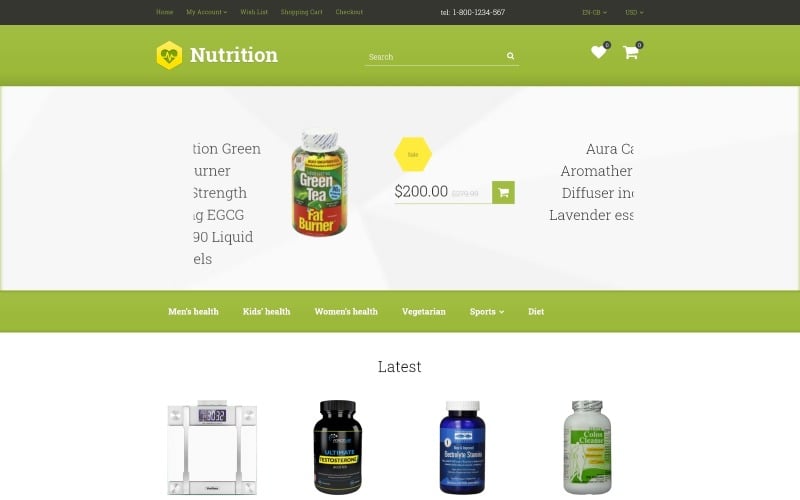This is a detailed screenshot of a website for the brand "Nutrition." At the very top, there is a black navigation bar featuring green text options, alongside a phone number displayed in white text. Below this is a green bar, carrying the same color scheme.

On the left side, not completely to the edge but slightly to the left, there is a distinctive logo consisting of a yellow hexagon with a cutout heart in the center, revealing the green background. A yellow heart rate monitor line cuts across the heart. The brand name "Nutrition" is prominently displayed in bold white text next to the logo.

Centered on the page is a search bar, and to the right are icons for a heart and a shopping cart, both in white. Each icon has a gray notification indicator showing "0."

Partially obscured by a white overlay is some text likely describing products. The visible content includes "green strength GCG liquid." An adjacent product image shows a can or bottle labeled as "Green Tea Fat Burner," featuring a green background and yellow text with a red backdrop. This product is priced at $200 and has a shopping cart option available.

Further mentioned is an "Aura Aromatherapy Diffuser Lavender," but this text is also partially obscured on the right side. 

Below, another green bar with white text options includes categories such as men's health, kids' health, women's health, vegetarian, sports, and diet.

Underneath this bar, four product images are displayed under the heading "Latest," written in black text. Three images are of small bottles in black, blue, and white colors, while the item on the far left appears to be a box with a time indicator.